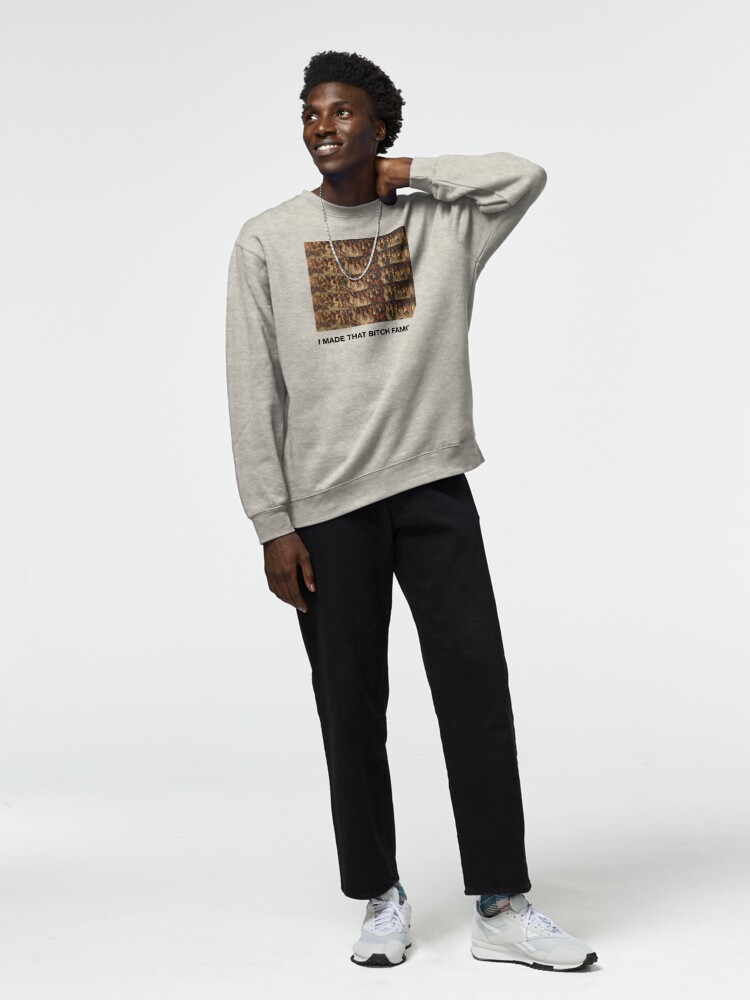The photograph is a color image featuring a young, clean-shaven Black man with short, curly black hair standing on a white floor against a light gray background. He is posing with his face turned towards the top left corner, while his body faces forward. His left hand is bent at the elbow, reaching behind his neck. The man is dressed in white tennis shoes with black soles; his left foot points to the right and his right foot points forward. His socks are plaid in blue, white, and red, partially visible due to his slightly short black pants that stop just above the ankle. He wears a gray long-sleeve sweatshirt with a brown square image on the front and black text beneath it that reads, "I made that bitch famous." Around his neck, he sports a silver chain necklace. The man is smiling slightly, completing the confident yet relaxed pose that suggests he might be a model in a photo shoot.